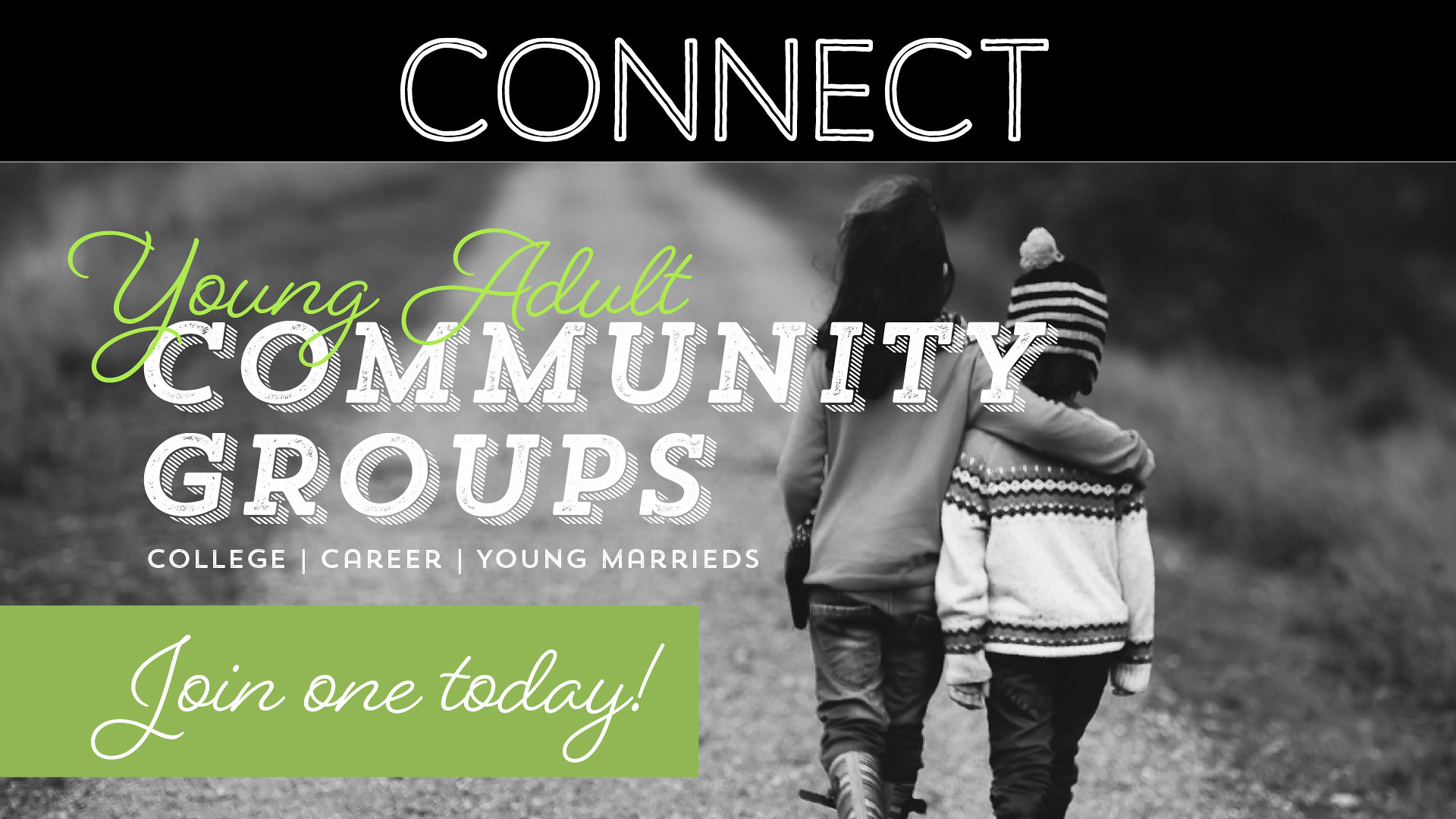The image is a detailed advertisement for a church group, featuring a black and white photo centered on a black border. At the top of the image, the word "Connect" is prominently displayed in bold white lettering. The photograph showcases a poignant scene of two children walking away from the viewer down a long dirt or gravel road. The taller child has their arm wrapped protectively around the younger child's shoulders. Both children are dressed warmly; the taller one is wearing a long-sleeve shirt, jeans, and what appear to be snow boots. The younger child is clad in a Christmas-style sweater and black pants, complemented by a snow hat with a pom-pom.

Overlaying the photo is a series of texts: "young adult" written in green cursive, followed by "Community Groups" in larger white text with a sketchy drop shadow effect. Below these main titles, smaller white lettering lists "college," "careers," and "young marrieds." At the very bottom, a green banner with white cursive text reads "Join one today."